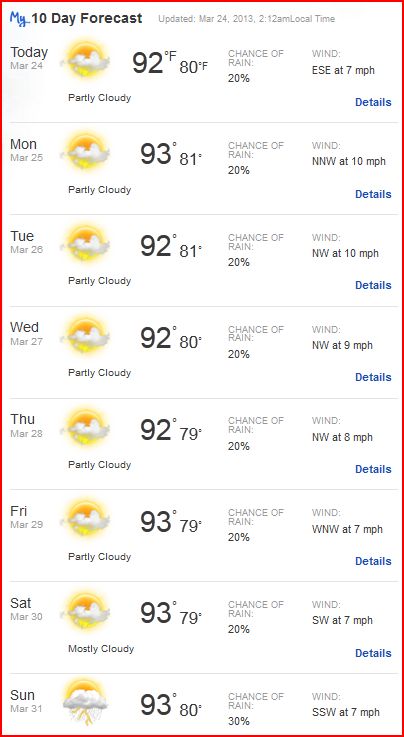Screenshot of a detailed 10-day weather forecast, updated on March 24, 2013, at 2:12 a.m. local time. The forecast spans from March 24 to April 1. Each day’s weather details are stacked vertically, including high and low temperatures, chance of rain, and wind direction:

- **Today, March 24**: Partly cloudy with a high of 92°F and a low of 80°F. There is a 20% chance of rain and winds coming from the east-southeast at 7 mph.
- **Monday, March 25**: Partly cloudy with a high of 93°F and a low of 81°F. A 20% chance of rain remains, with variable winds.
- **Tuesday, March 26**: Similar conditions with a high of 93°F and a low of 81°F. A continued 20% chance of rain.
- **Wednesday, March 27**: Partly cloudy, high of 92°F, low of 80°F with a 20% chance of rain.
- **Thursday, March 28**: Forecast predicts partly cloudy skies, a high of 92°F, and a low of 79°F, with a 20% chance of rain.
- **Friday, March 29**: Expect partly cloudy weather, high of 92°F, low of 79°F, and a 20% chance of rain.
- **Saturday, March 30**: Partly cloudy, high of 92°F, low of 79°F, and a 20% chance of rain.
- **Sunday, March 31**: Partly cloudy, high of 92°F, low of 80°F, with a 20% chance of rain.
- **Sunday, April 1**: Partly cloudy with highs of 92°F and a low of 80°F, but an increased rain chance of 30%.

Wind directions vary slightly throughout the forecast period, but the overall weather pattern remains consistent with partly cloudy skies and minimal precipitation.